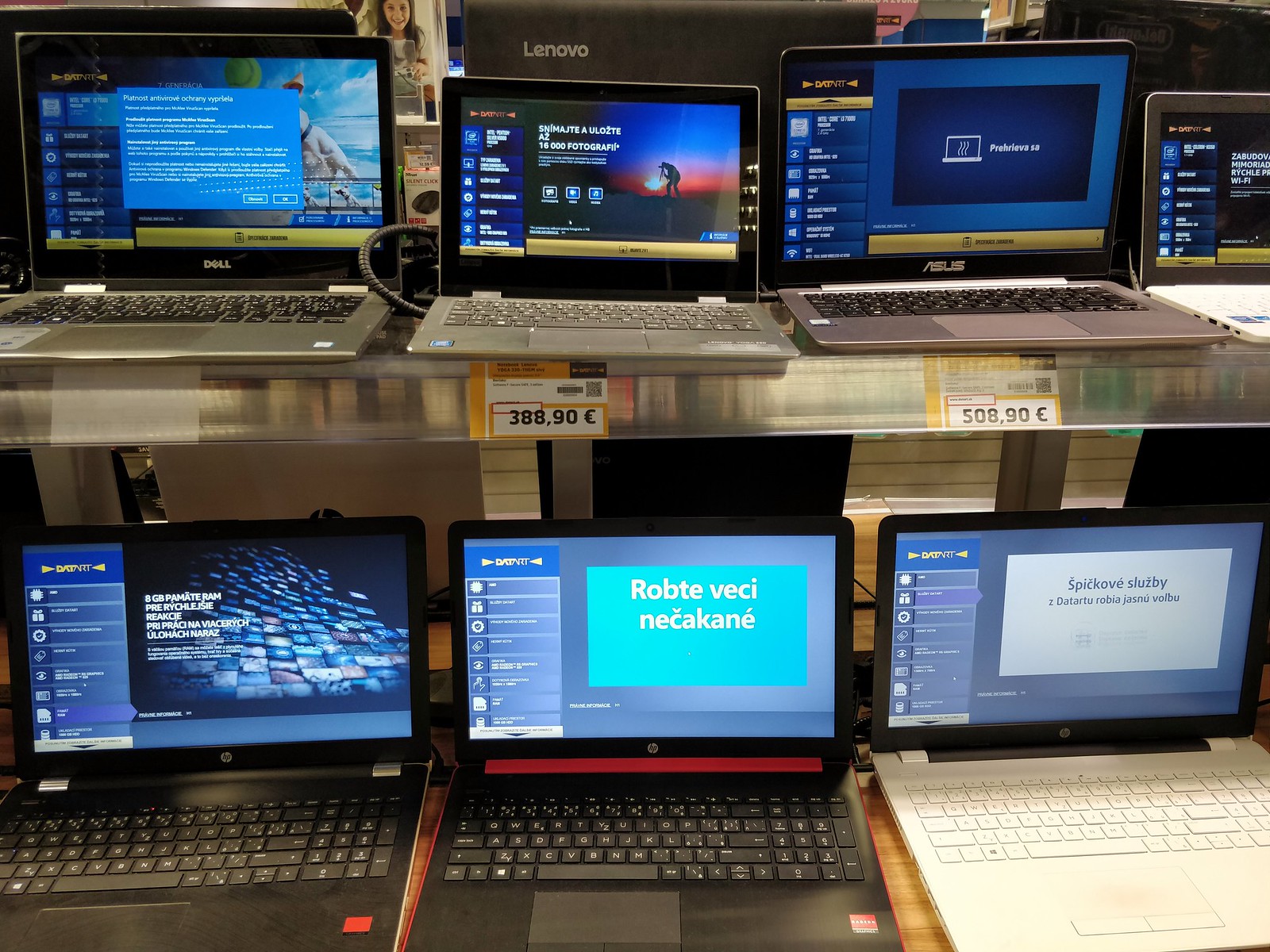The image depicts a sales display in an electronics store, showcasing a variety of seven laptops arranged on two clear glass shelves. The top row features four laptops, primarily silver with black bezels around the screens, except for one with a gray bezel. The fourth laptop on the top row is partially cut off on the right side of the image. The bottom row has three laptops, two of which are black with black bezels and one silver with a black bezel. Each laptop screen displays different images or text in various languages, possibly suggesting demonstration or test screens. Visible brand logos include Lenovo, Dell, HP, and Asus, with a large logo for Lenovo behind one of the displays. Price tags in euros are visible, indicating the laptops are for sale, and the overall presentation suggests that the laptops could be new or second-hand, but they are all operational.